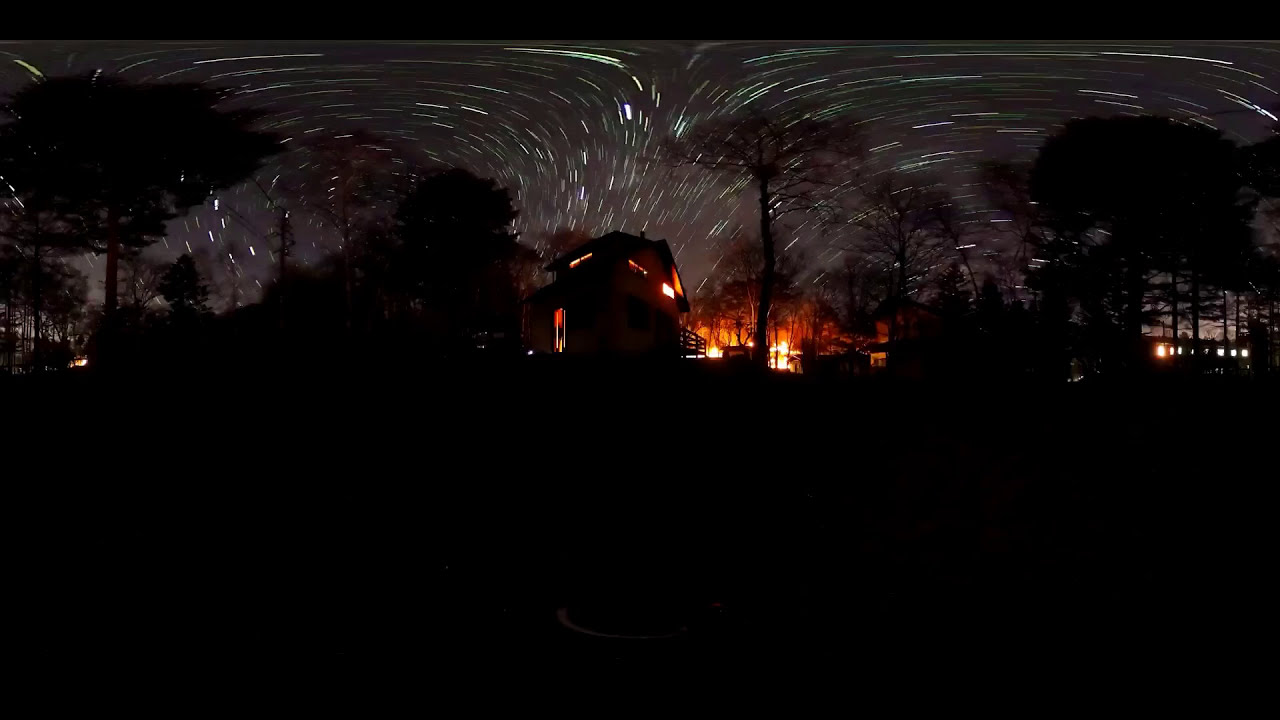This image captures an extreme 360-degree night-time scene, resulting in a highly distorted, split view that combines both sides of a residential area simultaneously. The photograph, taken with a time-lapse technique, displays the night sky filled with swirling, streak-like stars that arch across the darkness. Centered in the image is a house with soft, yellow-lit windows, backdropped by a star-speckled sky. The ground is cloaked in shadow, obscuring details but hinting at a grassy landscape beneath the darkness.

Off to the right side of the house, an orange blaze suggests an encroaching wildfire, casting an eerie glow on the surrounding trees and amplifying the night’s contrast. Scattered trees, some reflecting the fire’s light, punctuate the scene, adding texture to the dark environment. In the farther distance, a few streaks of light from what appear to be distant traffic or streetlights add layers to the depth. On the left side, a prominent tree and smaller distant trees frame the scene, their details blurred by the darkness. Despite the low light, the image conveys a vivid sense of a quiet residential area suddenly disrupted by the threatening presence of a wildfire.